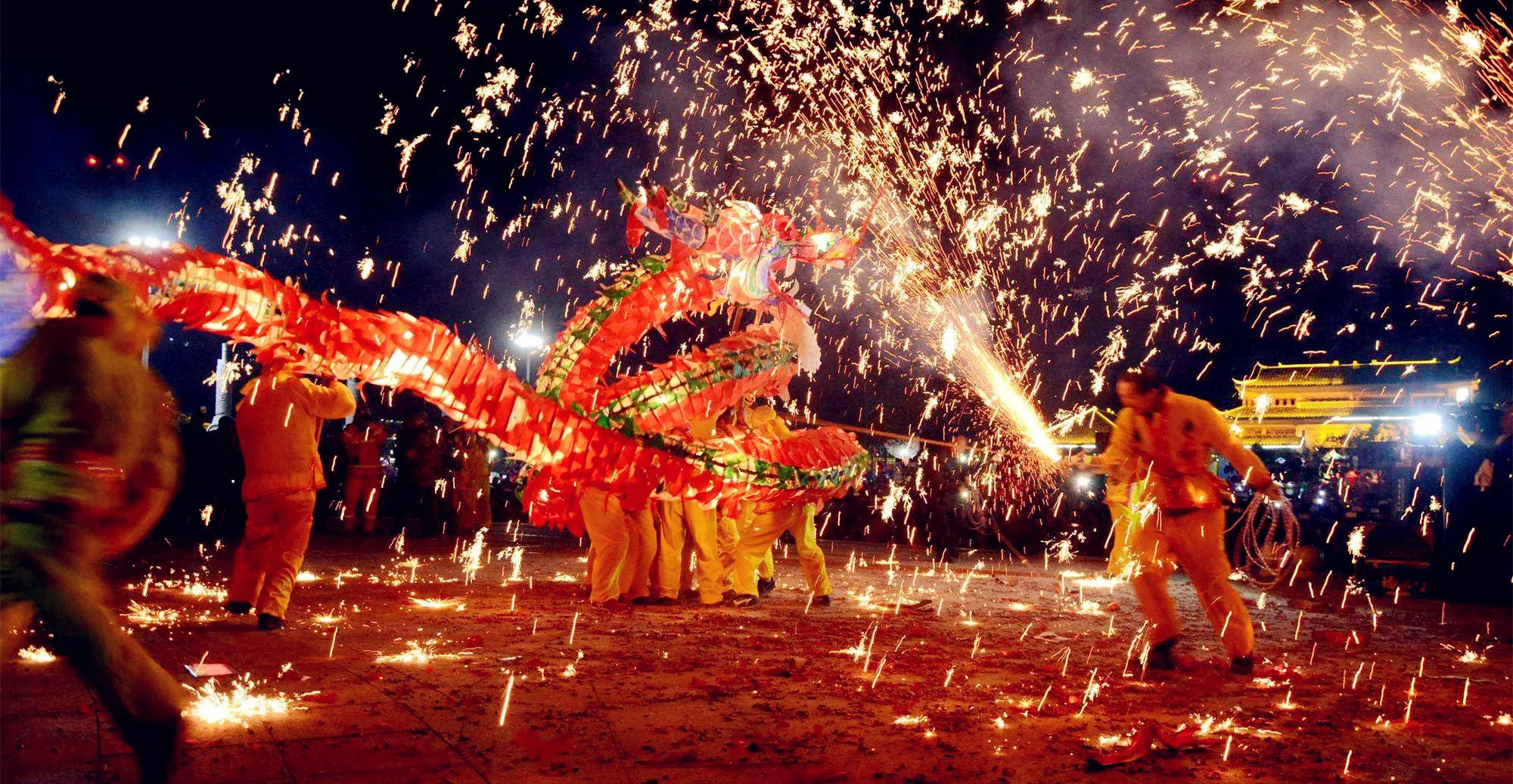The photograph captures a vibrant nighttime celebration, likely during the Lunar New Year. Central to the scene is a long, intricately decorated dragon puppet, about 30-35 feet in length, being skillfully maneuvered by several performers dressed in bright yellow jumpsuits. The dragon, primarily red with a striking green spine, is coiled up serpentine-like in the middle of the area, exuding a sense of dynamic motion. Its detailed head, adorned with horns and teeth, has its mouth agape, adding to the dramatic effect. 

To the right, a man launches fireworks, causing a cascade of sparks to illuminate both the dark sky and the performers below. The dragon itself also seems to be internally illuminated, making it stand out vividly in the night. Surrounding the performers, sparks fly and scatter across the ground, adding to the festivity's energy. In the background, you can glimpse buildings and a crowd of onlookers, all partaking in the spectacle of this well-decorated and lively cultural event.